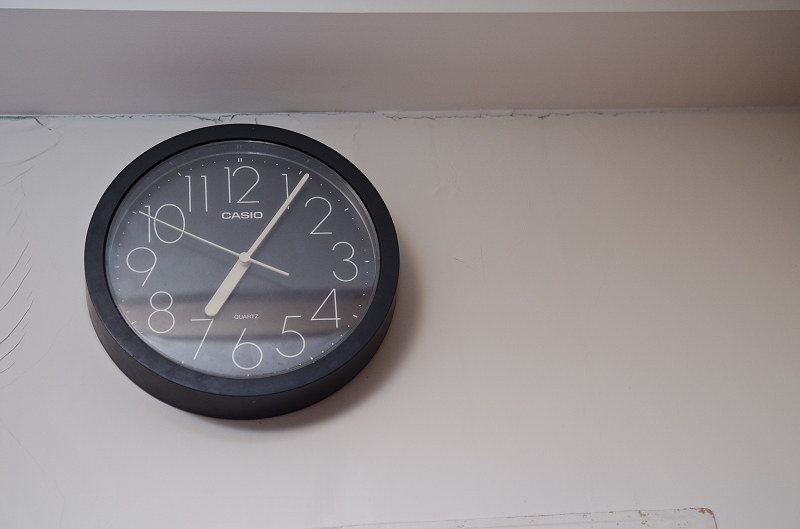The photograph depicts a black round Casio clock attached to an off-white, slightly cracked stone wall with a rough texture. Positioned to the left center of the horizontal frame, the image captures the upper portion of the wall where it intersects with the similarly rough and gray ceiling. The clock's face is adorned with a marshland and water design in grayish-blue and tan hues. The numbers, from 1 to 12, are prominently displayed in white, along with white hands: a short, paddle-shaped hour hand, a long, needle-shaped minute hand, and a thin second hand. Notably, the time shown is 7:06, with the hour hand on 7, the minute hand on the 1, and the second hand on the 2. Below the '12' is the brand name "Casio," confirming its make. The detailed cracks in the drywall emphasize the aged condition of the wall and ceiling.